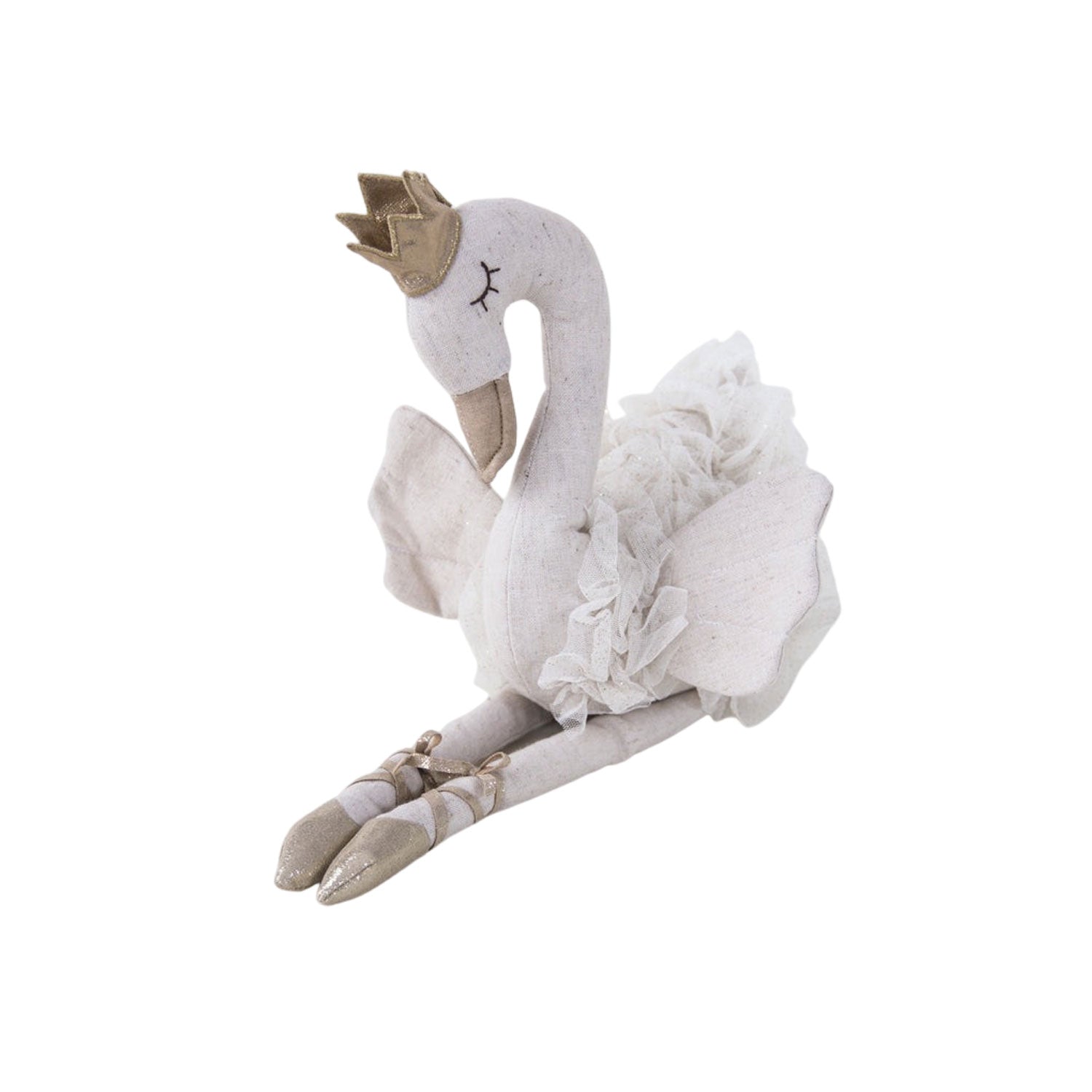This is a detailed photograph of a meticulously crafted stuffed swan made from a creamy white material with brown-tan specks. The swan features a tan-colored beak and a stitched black eye, complete with closed eyelids and delicate eyelashes. Adorning its head is a small, tan crown, adding a regal touch. The swan's back is covered in ruffled, fluffy cream-colored fabric, resembling a tutu, while its wings are a soft beige, fluttering angelically on either side. Its long, protruding legs are equipped with tightly fitted, golden glittery ballet slippers, each with tan ribbons tied in bows around the ankles. The swan is elegantly posed on a white sheet of paper, capturing an endearing and whimsical ballet-inspired aesthetic.